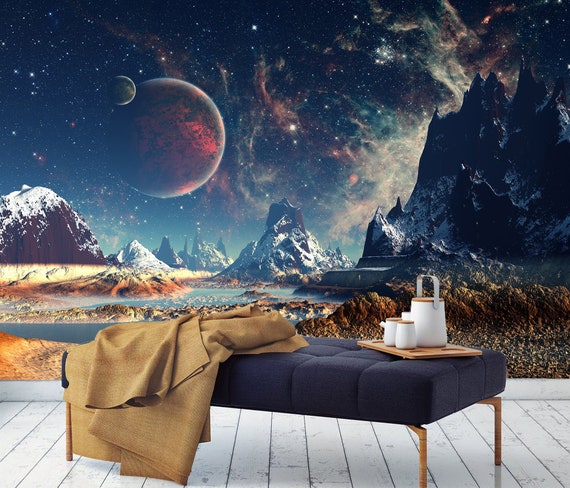In this digitally rendered image, the foreground showcases a sizeable footstool with a charcoal gray cushioned top and elegant gold legs. Draped over the footstool is a luxurious golden-colored blanket. Adjacent to this footstool, a wooden tray holds two pristine white cups adorned with a tan trim and a matching white pitcher featuring a handle and a tan lid.

The background of the scene transcends earthly boundaries, revealing an alien rocky landscape. Towering rock outcroppings exhibit a mix of white and earthy tones, while patches of water glint amidst the Martian-like terrain, painted in hues of brown, orange, white, and gray.

The celestial sky above enhances the otherworldly atmosphere with its breathtaking array of visuals. A canopy of deep black is scattered with white stars, interspersed with swirling pink clouds and variously colored planets, including pink and darker hues. The scene is further animated by several shooting stars, elevating the beauty of this cosmic tableau.